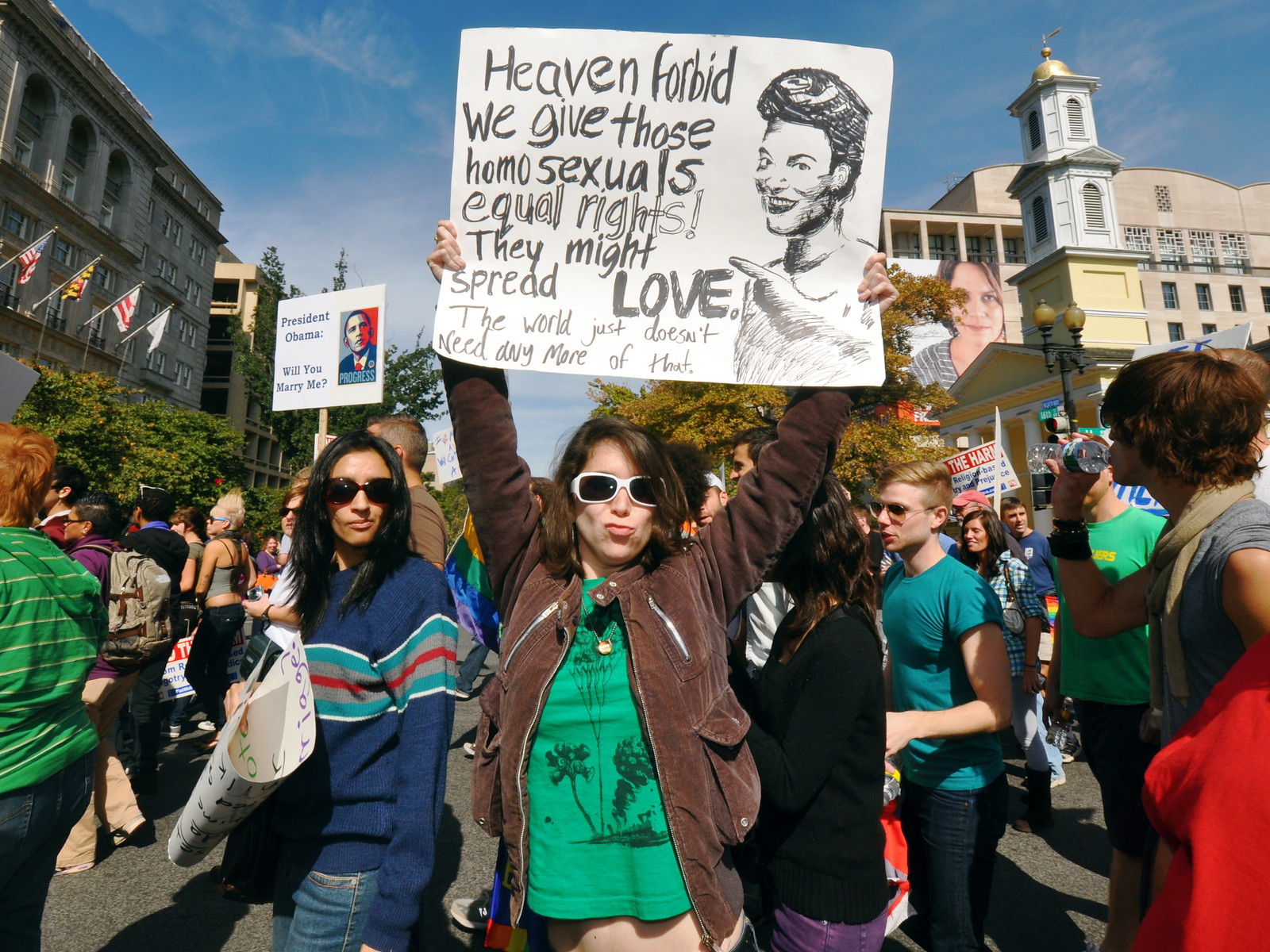This photograph captures a vibrant protest happening in a densely urban area, marked by a blue sky and flanked by tall, older buildings with diverse architectural features including arched windows and a prominent yellow building with a golden-domed tower. 

The diverse crowd, composed of young men and women in their 20s, is decked out in clothing of various colors, including red, green, blue, gray, purple, tan, and black. Among them, a woman in the center stands out. She sports a green t-shirt with a black logo, a brown suede jacket unzipped to reveal a bit of her midriff, and striking black and white sunglasses that frame her short brown hair. 

Her hand-drawn white poster features a black sketch of a person pointing towards the handwritten message: "Heaven forbid we give those homosexuals equal rights. They might spread love. The world just doesn’t need any more of that." Nearby, another protester raises a white sign illustrating a photo of Barack Obama with the text, "President Obama, will you marry me?"

The scene epitomizes the passionate atmosphere of the demonstration, underscored by the presence of flags of different countries and states, enhancing the sense of unity and diverse representation among the protesters.